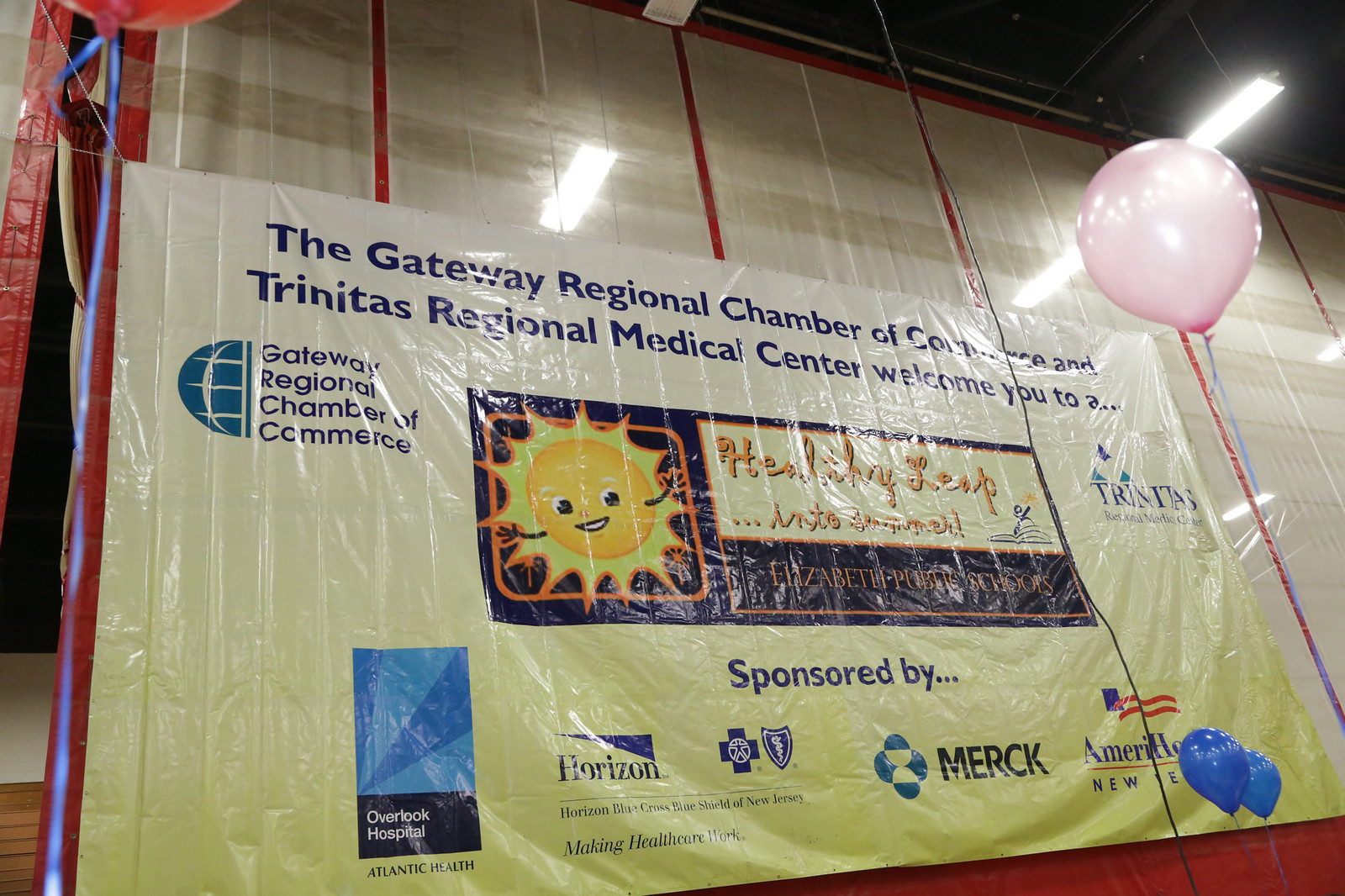The image showcases a photographic banner, presented inside a gym hall that features red stripes and other wall markings. The banner, seemingly made of a plastic-like material, transitions from a white background at the top to a light lemon yellow at the bottom. At the top, two lines of black text read, "The Gateway Regional Chamber of Commerce and Trinitas Regional Medical Center welcome you to a..." followed by an ellipsis. 

Dominating the center of the banner is a black insert featuring a cheerful sun graphic with a face and stick arms. To the right of the sun, in orange text, are the words "healthy leap into summer." Flanking this black insert on the left is the logo of the Gateway Regional Chamber of Commerce, depicted as a half-globe with accompanying text. To the right is the logo for Trinitas Regional Medical Center.

Below this central section, a smaller text reads "Sponsored By," followed by logos and names of several sponsors, including Overlook Hospital, Horizon Blue Cross Blue Shield of New Jersey (with respective Blue Cross and Blue Shield symbols), and Merck (depicted with blue and white balls). The lower portion of the banner is obscured by two dark blue balloons, and a prominent pink balloon is noticeable in the top right corner. The entire scene is accented by a fluorescent light shining onto the banner, causing some glare and reflections.